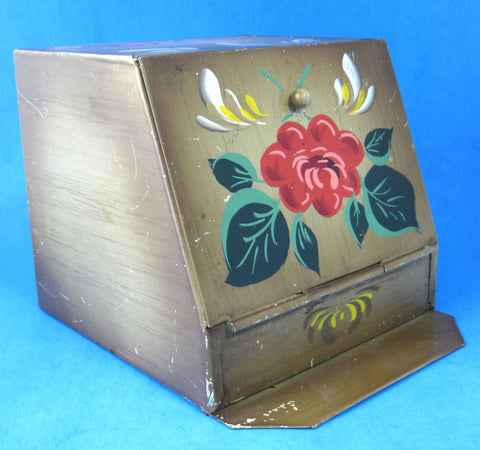This image features an antique wooden box with a unique pentagonal shape against a vibrant blue background. The box, resembling an old-fashioned bread box, has a slanted front panel that opens downward, indicated by visible hinges near the bottom. It has a small wooden knob handle situated above a central floral motif. The flower, painted in rich red hues with pink accents, is surrounded by dark green leaves with lighter green veins. Above the flower, delicate white and yellow swirls add an ornate touch. The lower portion of the box features additional floral patterns in yellow and darker colors. The box’s design and intricate artwork give it a timeless, vintage appeal.